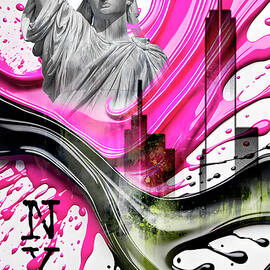In this abstract, collage-like painting set against a white background, vivid splashes and brushstrokes of black and bright pink dominate. The composition captures a silhouette of New York City with notable landmarks in grayscale. The lower half of the Statue of Liberty, from the nose to the chest, appears in gray—the green patina of reality replaced with a monochromatic tone. The Empire State Building and the World Trade Center with its antennas can be discerned in the mid and right sections. A dynamic, black stripe runs horizontally across the piece, branching down and to the right. Adding to the vibrant chaos, purple with maroon and red accents streaks above the black stripe, moving outward from the left. In the bottom left corner, distressed black lettering spells out "New York, NY," though part of the “Y” is cut off, and a dripped “C” hints at the word “City.” The painting exudes an energetic, almost frenetic quality, blending structured elements with spontaneous splashes and drips of color.